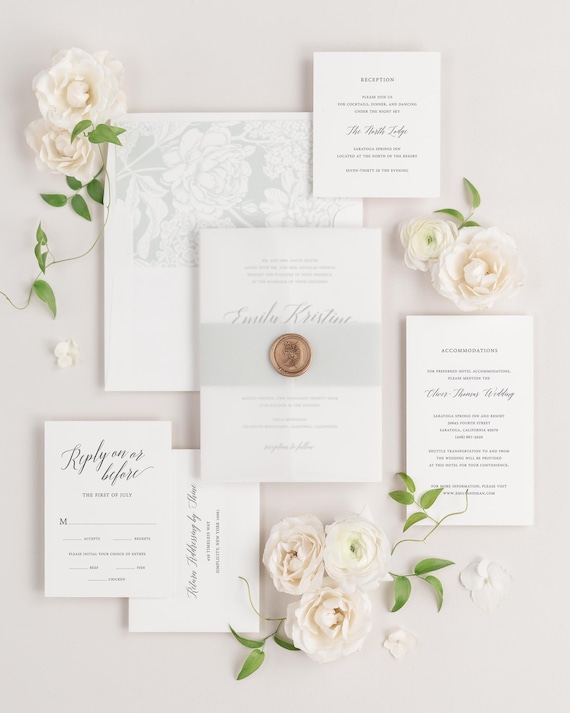This image, in a vertical rectangle layout, showcases a collection of overlapping wedding invitations and related stationery against a light gray background. Central to the image is a folded white invitation with engraved print, featuring the name "Emily Christine" elegantly displayed in cursive. This card is adorned with a gray band and a circular gold medallion. Surrounding this central piece are various other cards: an RSVP card, a reception details card, and an accommodations card, each with black text and cursive embellishments. A floral motif runs throughout the arrangement, with white roses and greenery interspersed among the pieces. Notably, an open envelope reveals an inner lining patterned with gray and white floral designs. The entire scene is imbued with a delicate and sophisticated ambiance, framed by strategically placed white roses and green leaves.